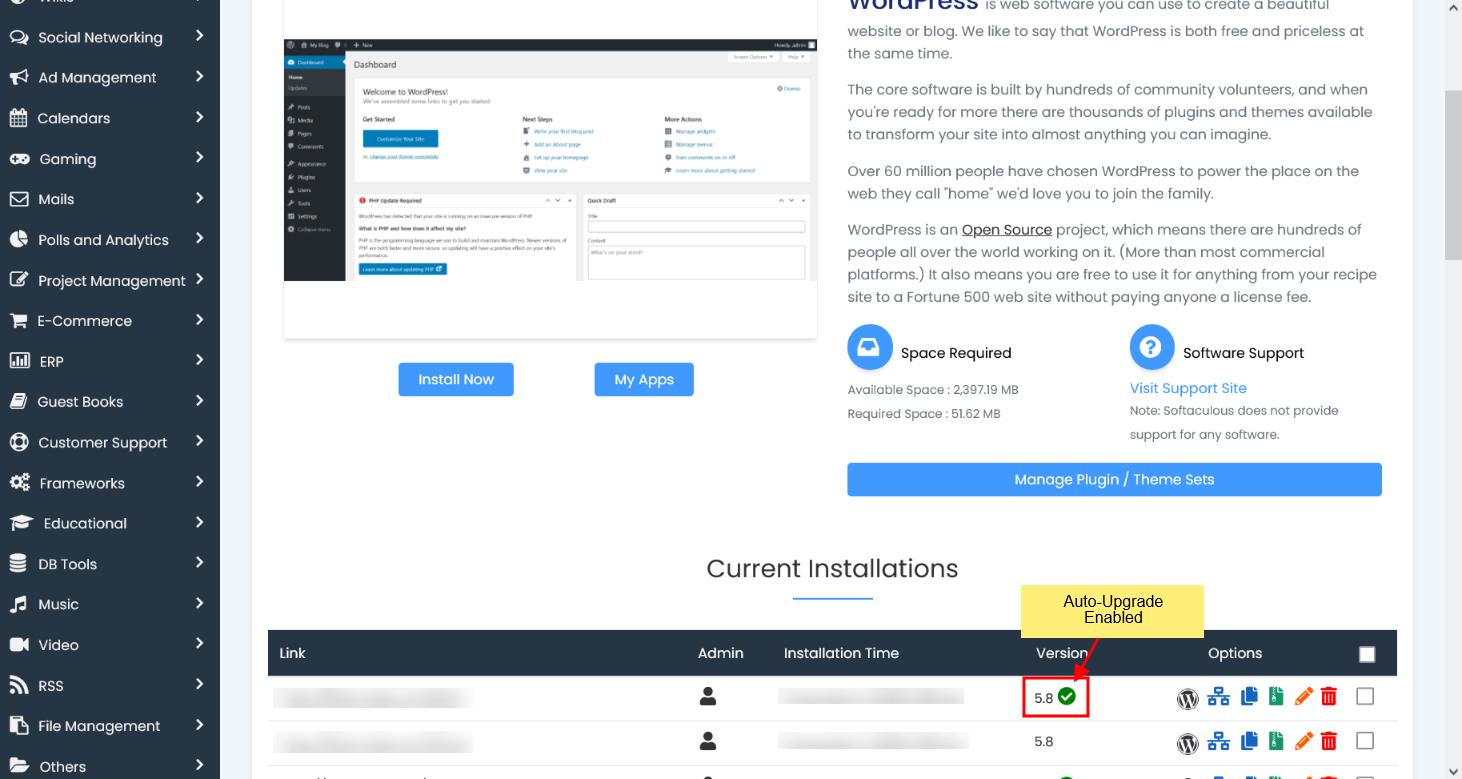The image depicts an administrative interface of a website builder or management tool, specifically resembling a WordPress admin page. The interface features a dark blue vertical navigation bar on the left side of the screen, containing a series of icons next to category names listed vertically. To the right of each category name, there is a right-pointing arrow indicating that the category can be expanded for more options.

The main section of the interface, which has a clean, white background, displays a pop-up window. At the top of the pop-up, the WordPress logo is prominent, accompanied by a brief description of the platform beneath it. The left part of the pop-up outlines essential details, such as the required space for installation and software support information. Below this, there is an option to "Manage Theme Sets."

To the right within the pop-up, a layout preview of the web page is shown, featuring buttons labeled "Submit Now" and "My Apps." Further down, there is an "Install Now" button, followed by a list titled "Current Installations" at the bottom of the page. This section includes an interactive panel displaying the details of currently installed themes or plugins, with a specific entry highlighted under the "Version" section. Above this highlighted entry, a note indicates that "Auto Upgrade" is enabled, ensuring that the installation stays up-to-date automatically.